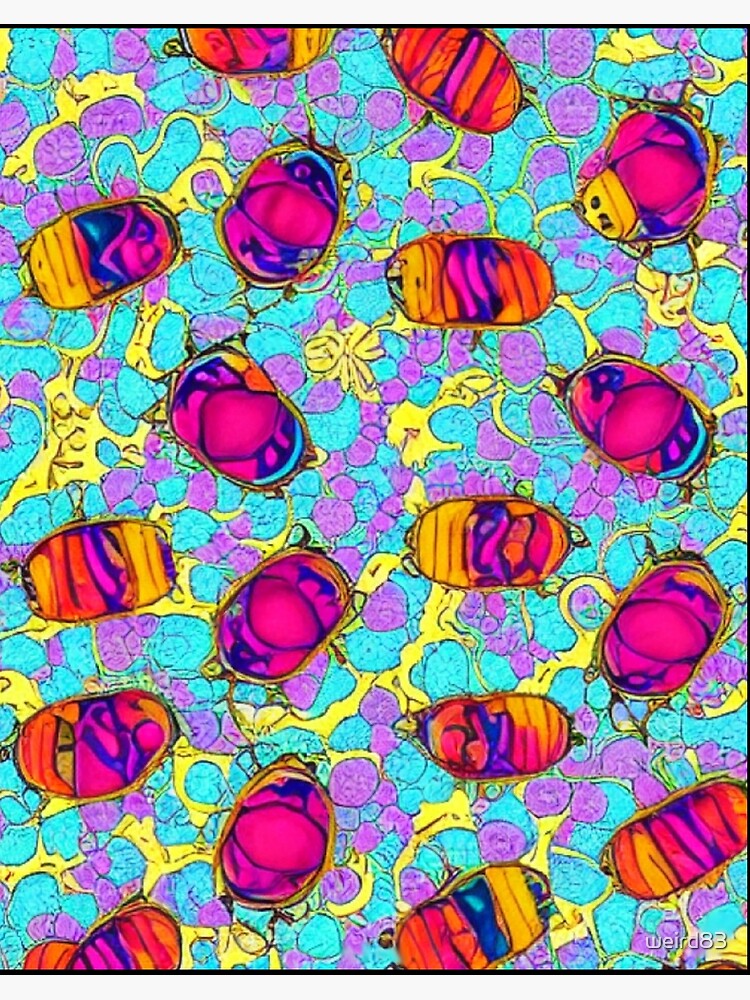The image is a vibrant, psychedelic artwork featuring what appear to be abstract, oval-shaped entities reminiscent of cellular molecules or beetles. These entities are predominantly colored in shades of pink, orange, purple, and blue and are scattered across the canvas in a seemingly random fashion. The background is a vivid mosaic of purple, blue, and yellow splotches, further adding to the chaotic, surreal aesthetic. Each oval shape is unique, adorned with varying patterns and colors, contributing to an overall sense of detailed individuality. Despite their beetle-like appearance, no legs or distinct appendages are visible, emphasizing the abstract nature of the artwork. The image is saturated with bright, over-the-top colors, making it a striking example of modern digital or painted psychedelic art.